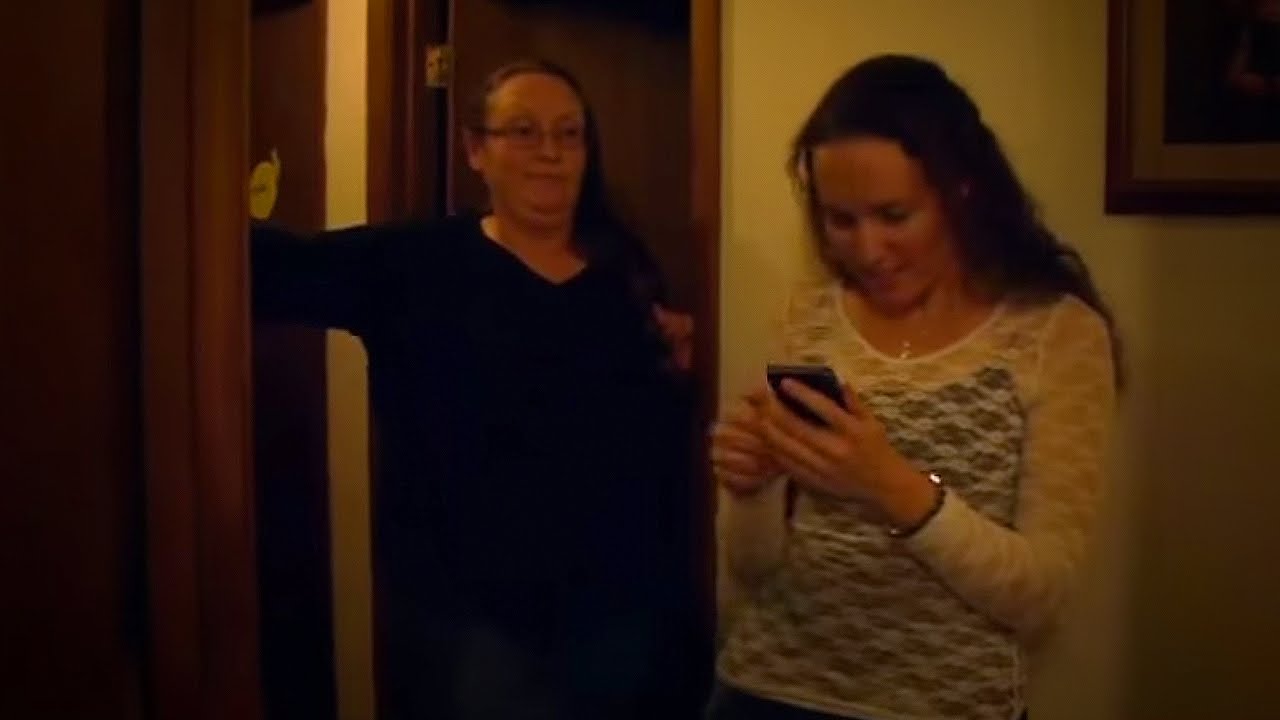In a dimly lit, orange-hued hallway, two Caucasian women with long brown hair are captured in a moment of interaction. The younger woman on the right, dressed in a white lace shirt layered over a black tank top, is engrossed in her smartphone, a smile of excitement spread across her face. A necklace adorns her neck, and a wristwatch or bracelet is visible on her left arm. Beside her, slightly to the left, stands an older woman, possibly her mother or sister, clad in a black v-neck top and glasses. She leans against a wooden doorframe, her left arm resting on the wall, watching the younger woman with a skeptical expression. The scene is framed by cream-colored walls, subdued by the dim light, and brown wooden doors and trim. The upper right corner of the image hints at a framed painting, adding a touch of homeliness to the setting.